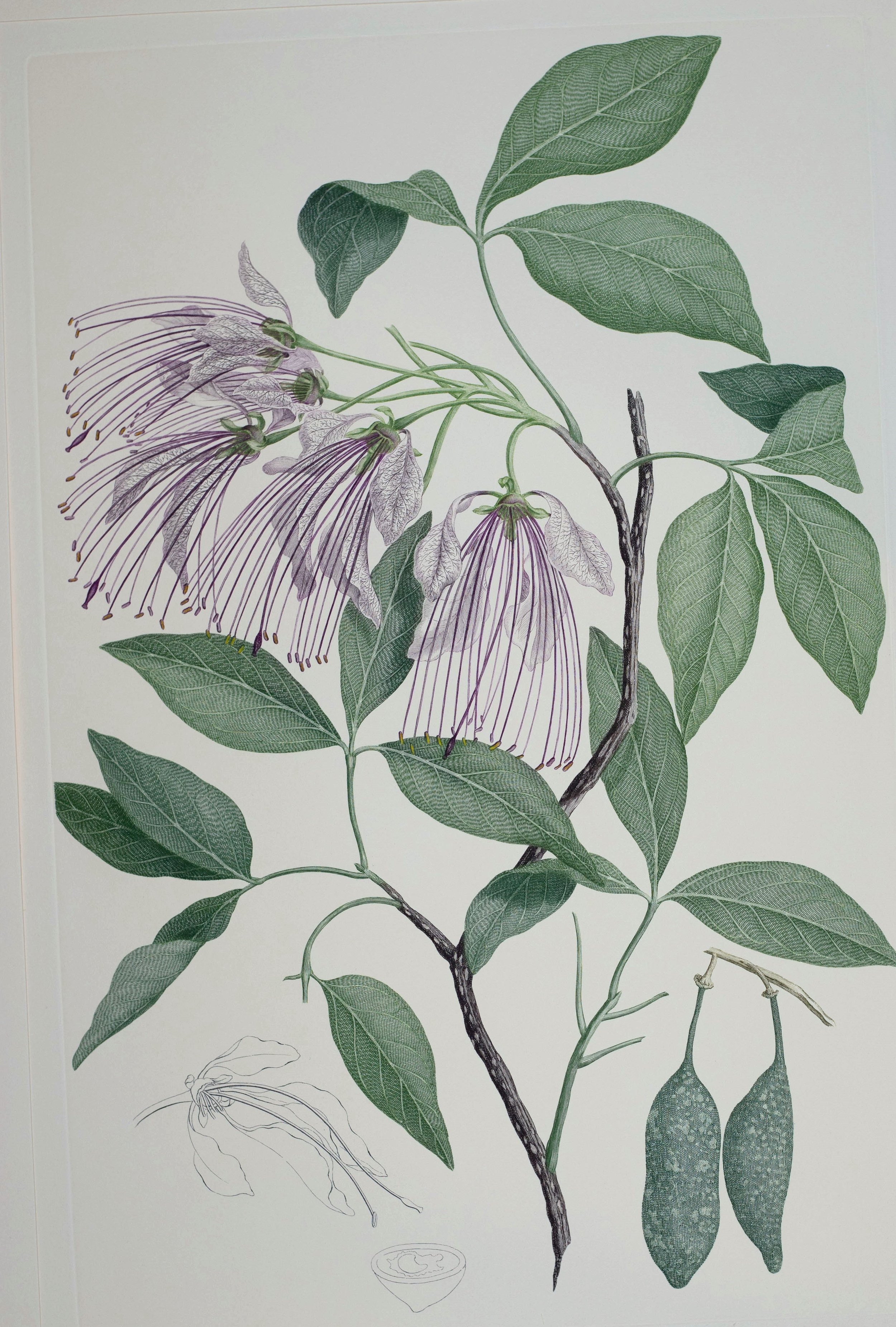This detailed illustration, likely from a botanical book, depicts a delicate, lacy branch section adorned with flowers and leaves. The branch, slender and thin, features pointed oval-shaped green leaves and flowers that hang downward like sheer skirts, with long, spindly purple stamens and translucent petals marked by purple lines. The flowers are suspended elegantly from the branch, which is not as thick as a tree branch, suggesting it is from a flowering plant or shrub rather than a tree. Set against an off-gray background, the illustration exudes the aesthetic and educational charm of classical botanical prints, designed to help identify different plants in nature. This piece, devoid of any additional elements like bugs or other flowers, presents a focused, detailed study of this exquisite and uncommon botanical specimen.